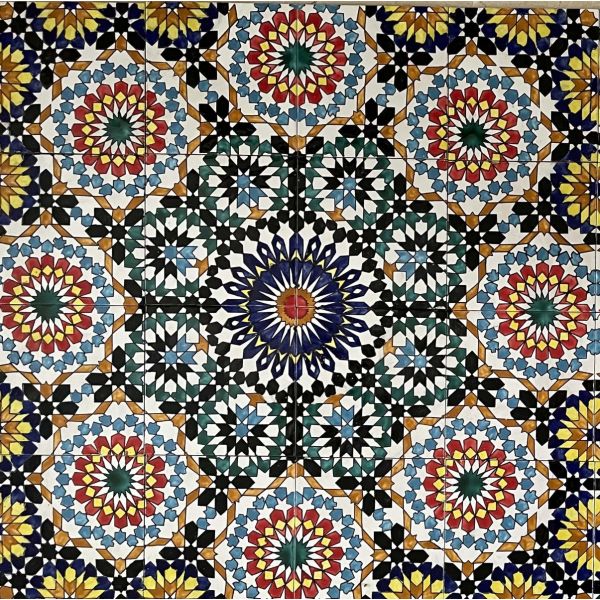The image showcases an intricate and colorful mosaic tile design, reminiscent of a kaleidoscope pattern with concentric circular arrangements. At the very center, there is a red circle with a yellow sunburst and white spikes, encircled by a blue, angular sunburst-like outline. Further out, blue tab-shaped tiles with pointed ends frame a central white diamond. Surrounding this, multiple circular patterns in white, black, blue, and green converge, bordered by brown diamond shapes. Moving outward, another concentric ring displays dark green, white, yellow, red, and blue hues embodying a flowery motif. Notably, there’s a golden eight-pointed star with blue baseball diamond-shaped tiles, red Monopoly-like house tiles with an A-frame roof, and yellow diamonds evolving into white star-like lights nestled within green tones. The outermost edge features yellow flowers encircled by small black blooms, layered with greenish flowers with red interiors and additional yellow accents. Overall, the design emanates a kaleidoscopic and floral aesthetic with a vibrant and detailed visual complexity.